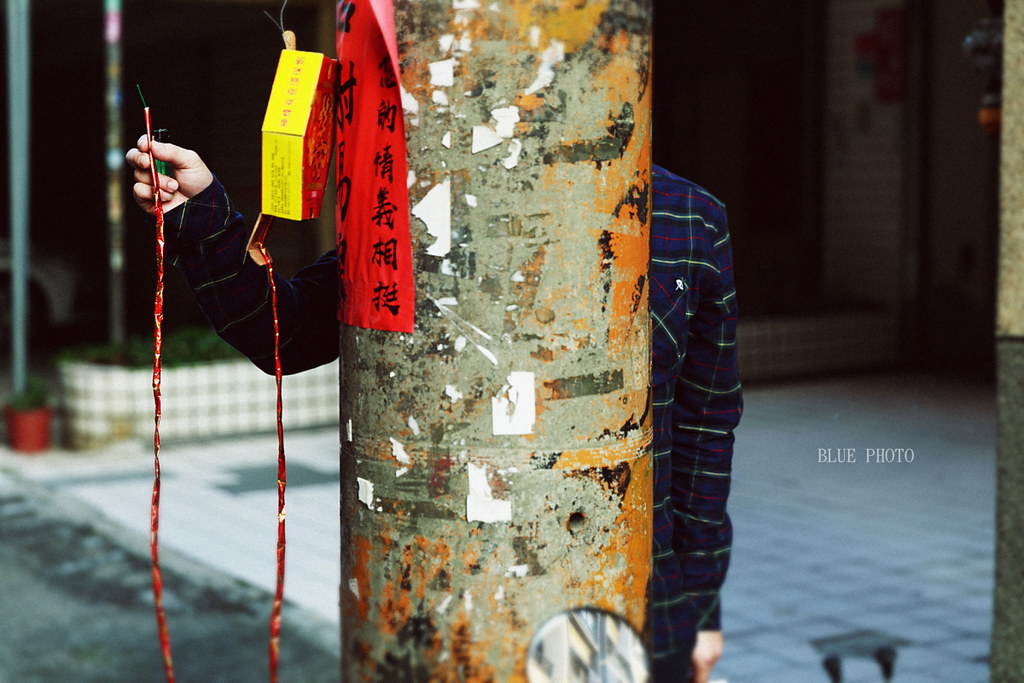The image depicts a scene in what appears to be an Asian country, characterized by a large stone pillar plastered with numerous torn-off paper pieces and a prominent red poster featuring Chinese writing. Hanging from the left side of the pillar is a red and yellow box that resembles a firecracker box, with a large red rope or fuse attached to it. Behind the pillar stands a man, though only his right shoulder, left arm, and hands are visible. He is attired in a flannel shirt with blue, red, and yellow stripes. In his hand, he ominously holds the end of the firecracker fuse along with a lighter, suggesting an imminent action. The background of the photo is largely blurred, revealing just enough to discern a pavilion area with tile work, a potted plant, some shrubbery, and dark shadows enveloping the scene. A watermark stating "blue photo" is visible on the right side of the image.